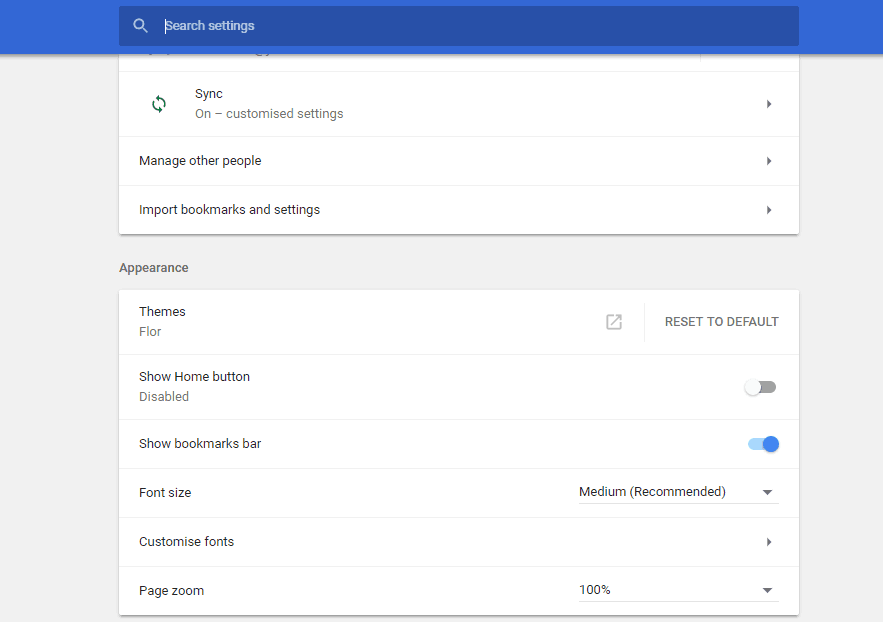This screenshot captures a browser window featuring a blue header, prominently displaying a search bar with a cursor in place and a magnifying glass icon on the left. The web page itself boasts a light grey background and is divided into two main sections.

The first section, titled "Sync," contains three rows: 
1. "Sync" with customized settings indicated by an icon of two arrows circulating in a circular fashion.
2. "Manage other people."
3. "Import bookmarks and settings."

Below this, the second section is labeled "Appearance" and includes multiple configuration options:
1. "Themes," which is currently set to "Floor," with an adjacent "Reset to default" option.
2. "Show home button," which has been disabled, as indicated by the untoggled switch on the far right.
3. "Show bookmarks bar," which is toggled on.
4. "Font size," set to medium, available via a dropdown menu.
5. "Customize fonts," currently blank.
6. "Page zoom," neatly set at 100%.

Overall, the screenshot meticulously captures the detailed settings and customization options available within the browser's user interface.